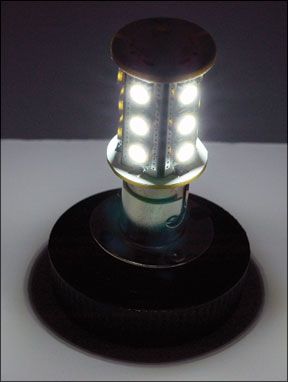This image, captured in portrait orientation, features a vintage lantern illuminated brightly as the main focal point. The lantern, resting on a white table, has a structure composed of both a metallic base and a top piece that appear to be copper or bronze in color. The lantern emits light through six small circular openings—three on each side—producing an intense, pure white glow that overshadows much of the surrounding environment. The narrow connection between the lights and the base is marked by a distinct white area. This strikingly illuminated lantern is set against a predominantly dark background with hints of gray and black, making the light source the central element of the composition. The image resembles a carefully staged photograph, potentially for showcasing or selling the lantern.